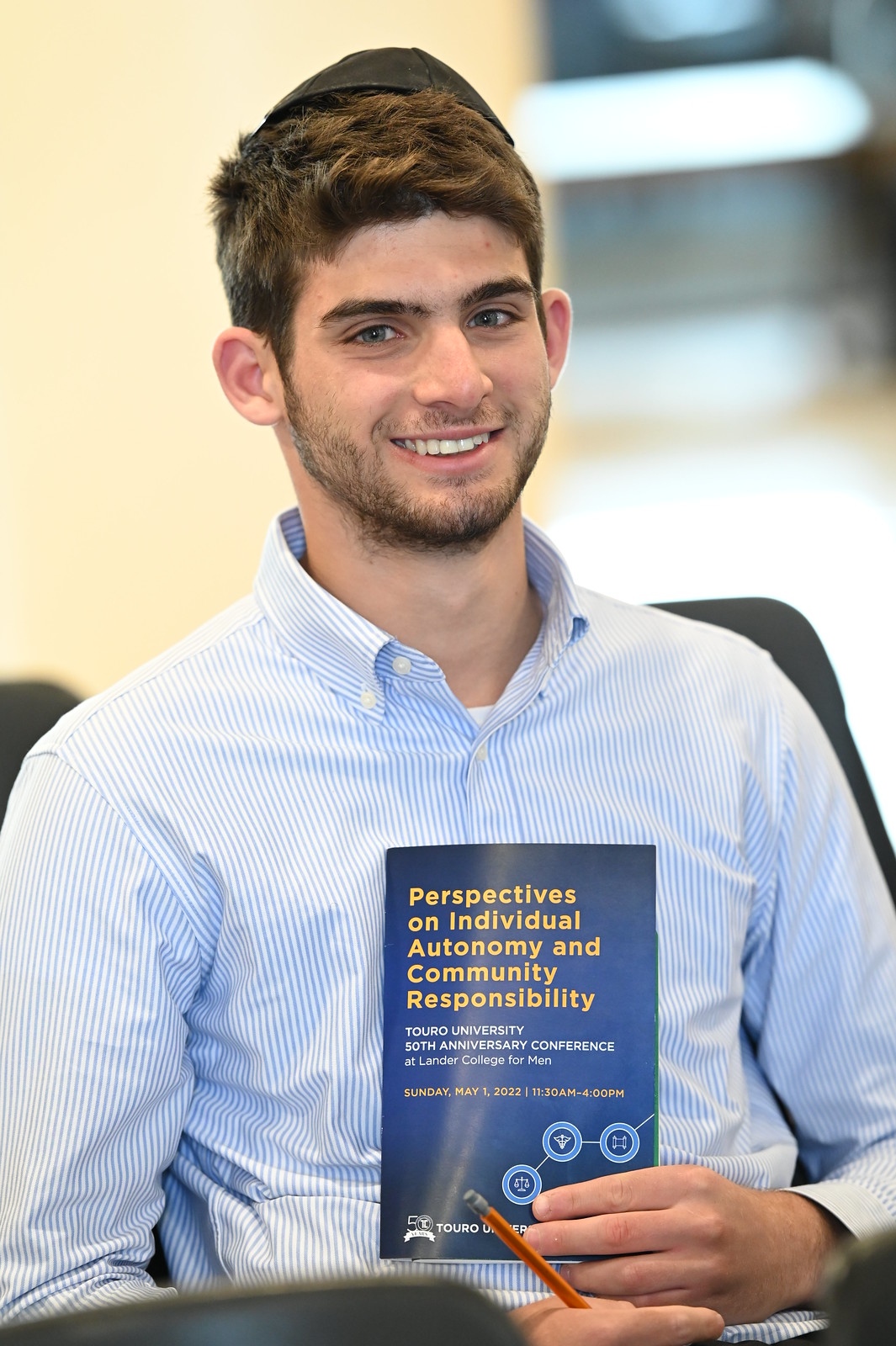In the photo, a young man, likely in his early 20s, sits smiling broadly at the camera. He has dark brown hair, blue eyes, and is wearing a black yarmulke. His facial hair includes a light, close-shaven beard and a sparse mustache. Dressed in a white and blue pinstriped, long-sleeve button-down shirt, he holds a dark blue book with yellow lettering titled "Perspectives on Individual Autonomy and Community Responsibility," with additional text in white and yellow detailing an event: "Truro University 50th Anniversary Conference at Lander College for Men. Sunday, May 1, 2022, 11:30 a.m. to 4 p.m." In his other hand, he grasps an orange mechanical pencil. The background is a blurry, cream-colored wall, providing no specific context to his location.